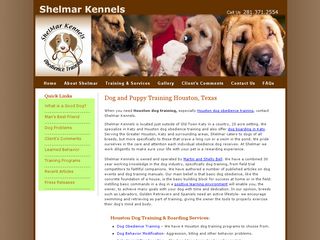This rectangular image features a brown border on both the left and right sides. In the center, the image showcases a business named Shelmar Kennels. 

In the upper left corner, the business name "Shelmar Kennels" is clearly visible. On the upper right corner, there's an illegible phone number, but the word "call" can be made out.

Below these headers are three photographs of dogs, arranged from left to right. The first image on the left is an illustration of a beagle-style dog enclosed in a circle, accompanied by the text "Shelmar Kennels" above it. To the right of this illustration, the first photo depicts a German Shepherd gently nudging a small tabby cat. Following that is an image of a tan-colored Cocker Spaniel with a human figure above it. The last photo on the far right is a close-up of a brown dog.

Beneath these photos is a brown banner with partially illegible text, from which a few words can be discerned, including "training," "services," and "contact." Below the banner, set against a white background, is brown text that reads: "dog and puppy training Houston, Texas."